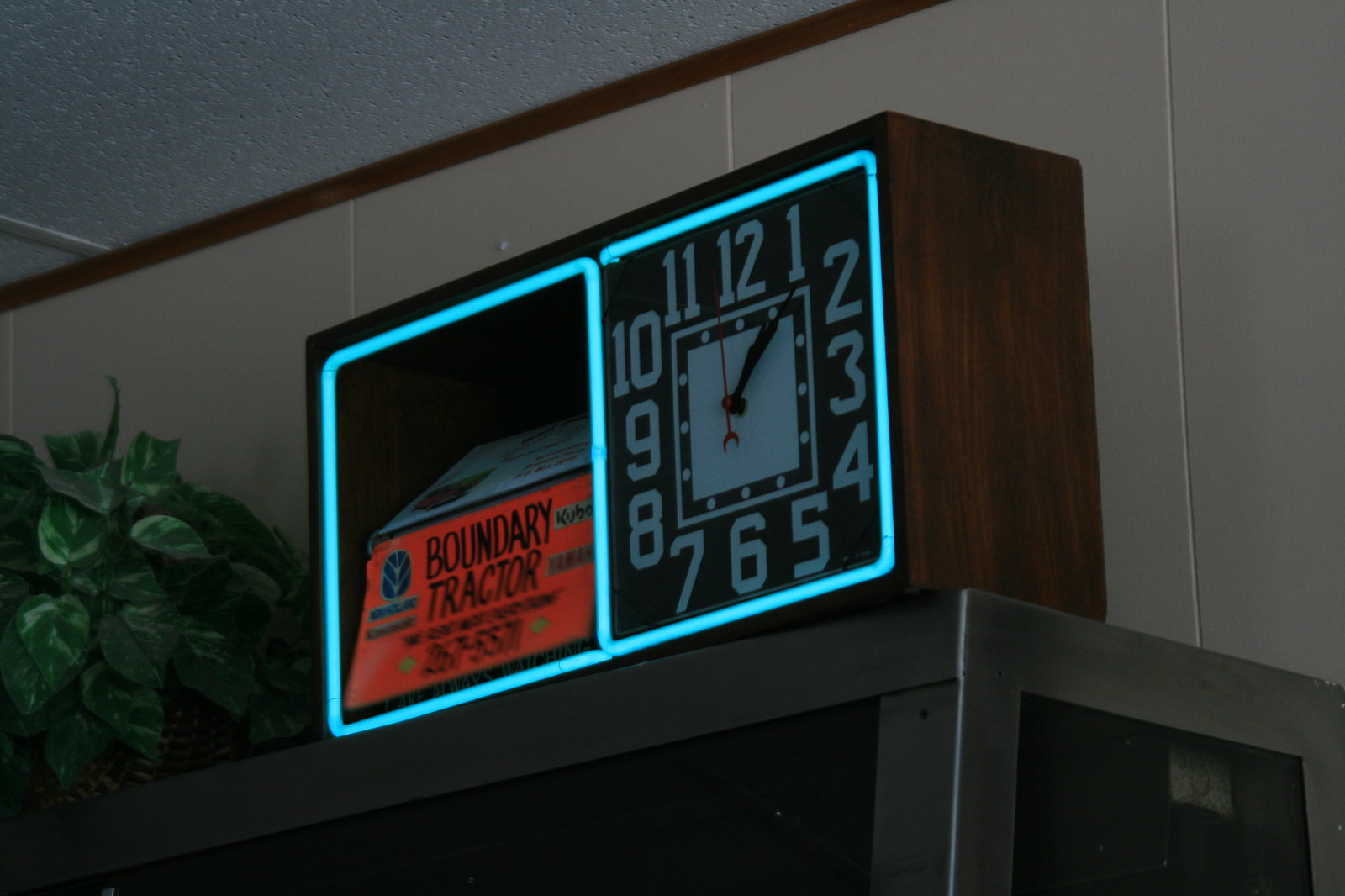A color photograph captures the corner of a room featuring a clock positioned on a cut-off gray metal shelf. The room has a tan-colored panel wall with a dark brown trim near the white drop ceiling. On the metal shelf, a wicker basket containing a green leaf plant is visible. The clock itself, a rectangular dark wood box, is divided by a blue neon LED border that separates it into two sections. The left side displays an orange sign with black text that reads "Boundary Tractor 2675571," along with a white paper above it that seems partially obscured. The right side features a black clock face with white numerals indicating hours 1 through 12, black minute and hour hands, and a red second hand with a small crescent moon shape at its base. The clock sits high, near the ceiling line adorned with thin brown molding, blending well with the room's cream-colored walls and industrial aesthetic.